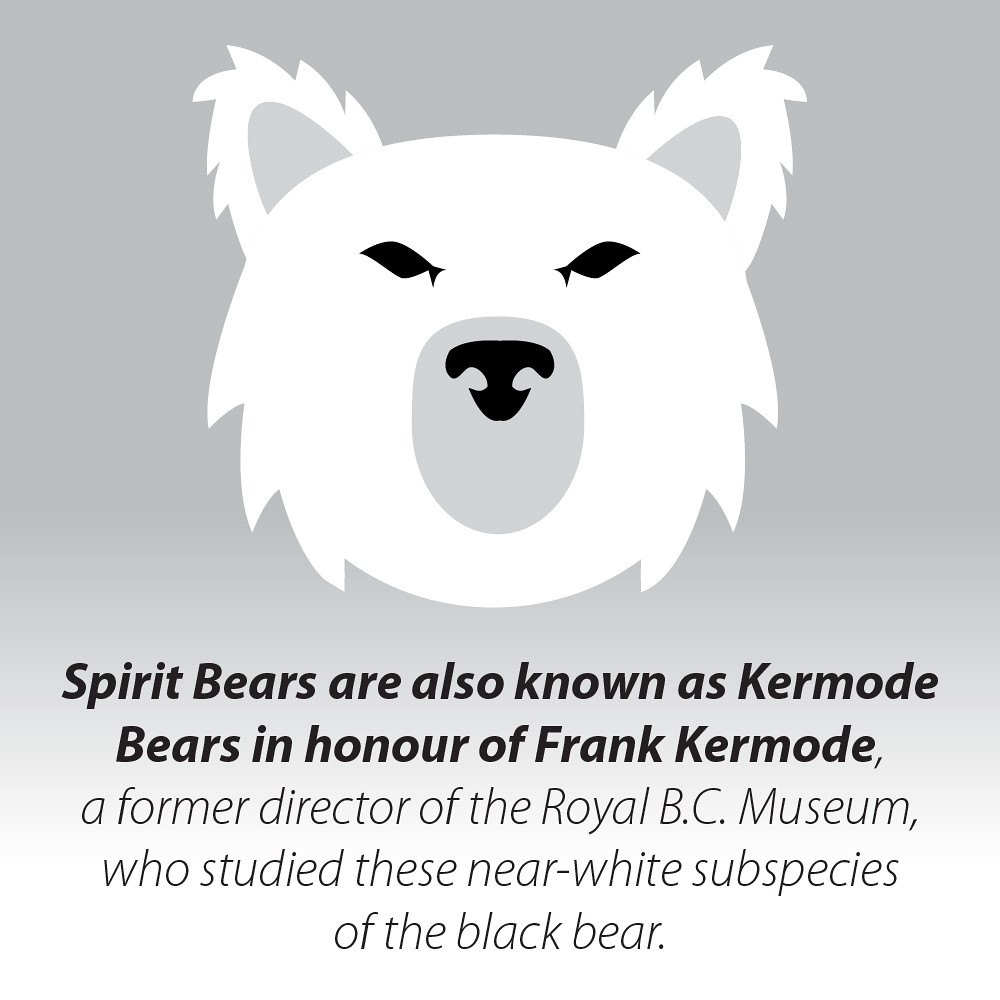The image features a graphic design on a poster with a gradient background that transitions from dark gray at the top to white at the bottom. Dominating the upper half of the poster is an animated, 2D depiction of a bear's face. The bear's face is primarily white with slightly jagged edges to represent fur, and has distinct features including black eyes that appear somewhat menacing, a silver-gray snout with a black nose, and ears with gray centers.

Below the bear's face, in bold black text, is the statement: "Spirit bears are also known as Kermode bears in honor of Frank Kermode." Following this, in regular black text, the poster continues: "A former director of the Royal BC Museum who studied these near-white subspecies of the black bear." The overall design emphasizes a clean and informative layout, providing both a striking visual of the spirit bear and concise educational information about the species and its connection to Frank Kermode.